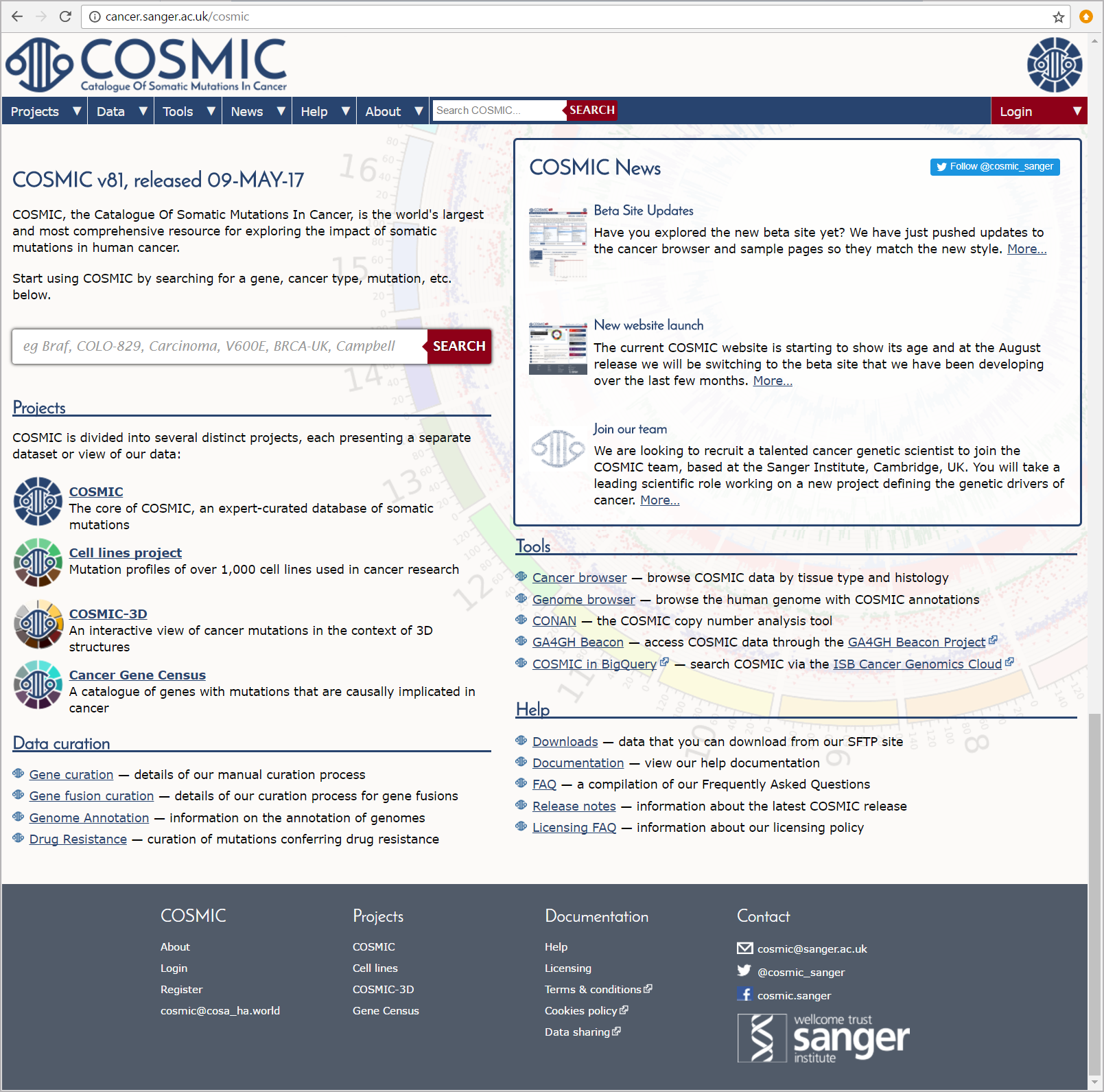This detailed caption provides a comprehensive description of the Cosmic website, particularly focusing on the user interface and its elements:

---

The image features the homepage of the COSMIC (Catalogue of Somatic Mutations in Cancer) website, accessible via the URL cancer.sanger.ac.uk/cosmic. At the top left corner, the website prominently displays the name "COSMIC" along with the tagline "Catalogue of Somatic Mutations in Cancer." 

Occupying a prominent position at the top of the page is a blue navigation bar with several dropdown menus for "Projects," "Data," "Tools," "News," "Help," and "About." In addition, there is a "Search COSMIC" bar coupled with a red search button.

On the far right side of the navigation bar is a red "Log In" button, which also features a dropdown menu option. 

Situated on the left side of the main content area, the page displays "COSMIC V81," indicating version 81, followed by the release date, 9 May 2017. The text elaborates that COSMIC is the world's most extensive and detailed source for researching and understanding the somatic mutations found in human cancers. 

The main section invites users to start utilizing COSMIC by searching for genes, cancer types, mutations, and more using the provided search bar paired with another red search button.

Additionally, the page introduces different projects within COSMIC, explaining that the database is divided into multiple distinct projects, each offering unique datasets or perspectives. It highlights "COSMIC," the core section of the database containing expert-curated somatic mutations, and the "Cell Line Project," which profiles mutations across over a thousand cell lines used in cancer research. 

---

This caption not only describes the visual elements of the webpage but also provides insight into its functionalities and the resources available to users.